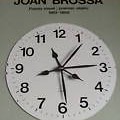This is a small image of an unusual analog clock with a white face and black markings, set against a gray background. The clock features an extraordinary design, having six hands instead of the typical two or three. These six hands are all the same length and style, with three pairs looking identical. The hands are pointing in various directions: between 1 and 2, 3, between 4 and 5, between 5 and 6, between 8 and 9, and between 11 and 12. Centered above the clock, partially cropped, is some black text that appears to say something like "Joe Bronson" or "Joan of Bronson," but it is difficult to read. There are also two smaller lines of text below the main heading, but they are too small and blurred to decipher. The bottom edge of the clock is also cropped out of the image. The overall impression is of a compact, square image displaying a puzzling timepiece.